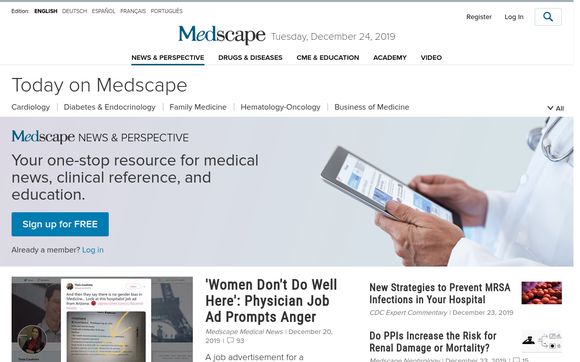This is a detailed caption for the given image:

"This screenshot from the desktop version of the medical website Medscape showcases its user-friendly interface and content-rich design. The Medscape logo prominently occupies the top of the screen, adjacent to the date displayed as Tuesday, December 24, 2019. On the top left, users can easily change the website’s language, with options available in English, German, Spanish, French, and Portuguese. The top right corner features a search button and options for user registration or login.

The website's layout is clean, with a predominantly white background. Below the logo, a navigation menu offers access to various sections of the site. 

Centrally placed is a main promotional image of a medical practitioner holding a tablet and a stethoscope, accompanied by an overlay of text on the left side that reads, 'Medscape, News and Perspective, your one-stop resource for medical news, clinical reference and education.' Beneath this text is a call-to-action button inviting users to sign up for free or log in if they are existing members.

Further down the page, the website features additional clickable images and links to news stories and articles. On the left, there is an image, although its text is too small to read in this screenshot. The center column highlights an article titled 'Women Don't Do Well Here', providing a link to the full story. The right side features two more links to articles, each accompanied by thumbnail images.

Overall, the website's front page resembles the layout of a newspaper, with the date at the top and various news stories displayed below, creating a comprehensive and accessible resource for medical professionals and enthusiasts."